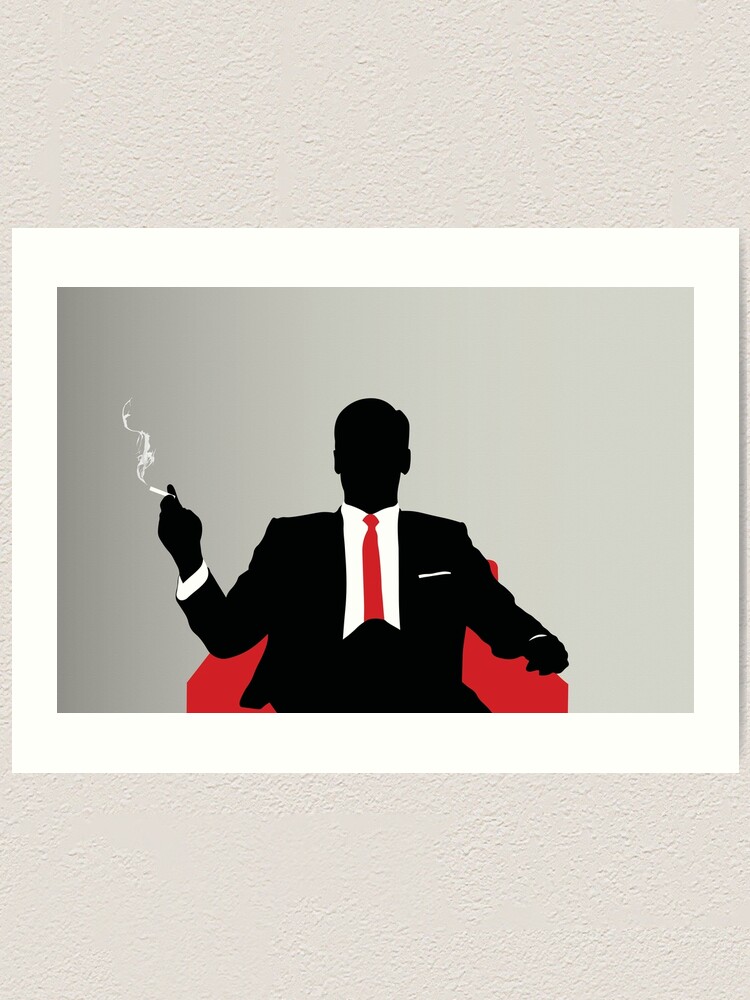The graphic masterfully portrays a silhouette reminiscent of Don Draper from Mad Men, seated in an orange chair. Clad in a black suit with a white shirt and an orange tie, the figure’s hands and face are obscured in darkness, adding to the silhouette effect. He holds a cigarette in his right hand, with a smoke trail elegantly rising from it. His crisp white shirt cuff peeks out from his suit sleeve, and a white handkerchief is neatly tucked in his left breast pocket. The background transitions from a darker gray on the left to a lighter gray on the right, framed by a thick white border. This graphic rests on a textured, eggshell-colored surface, creating a striking contrast.